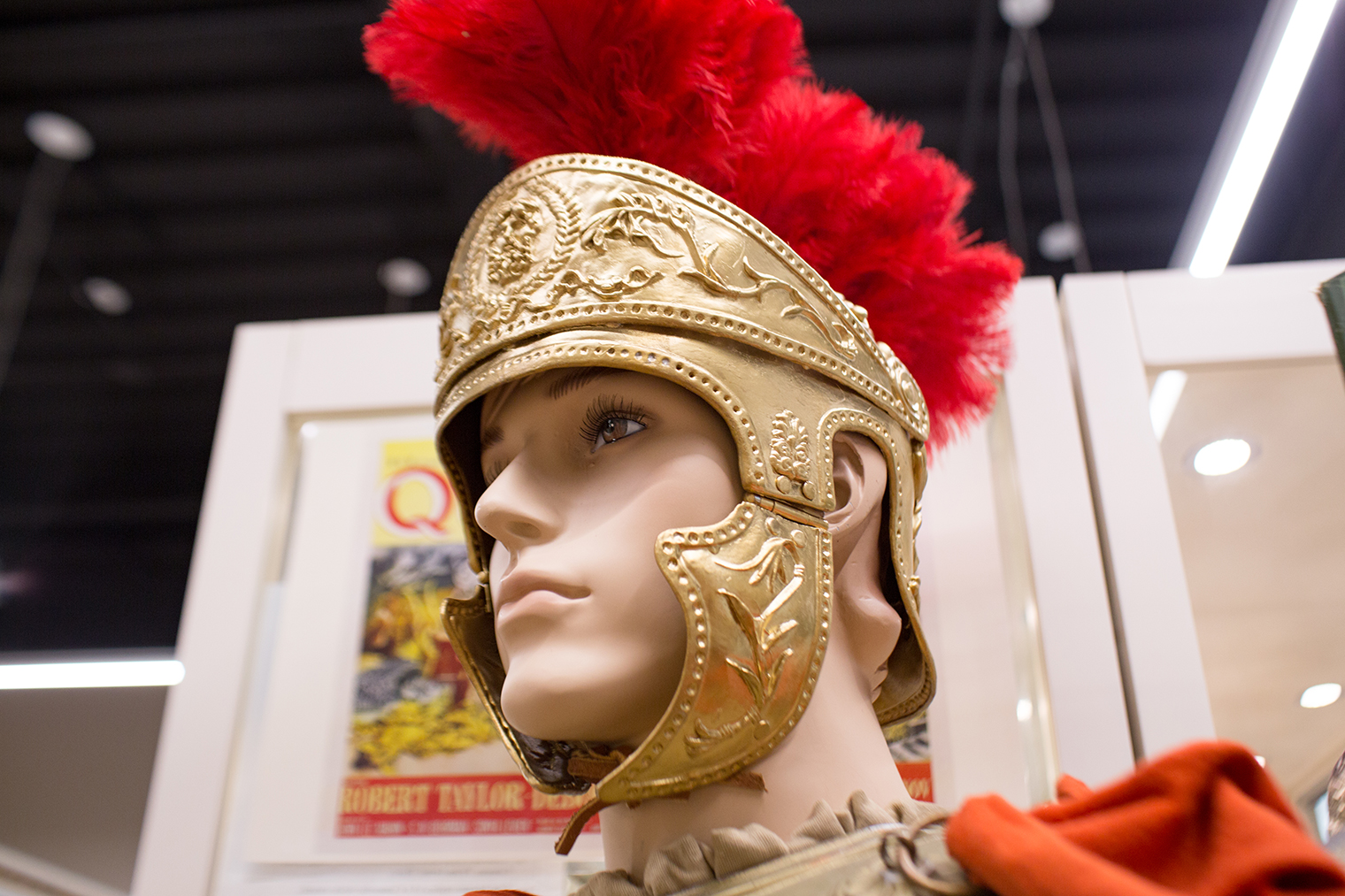This is a detailed color photograph of a mannequin dressed as a Roman soldier. The mannequin is adorned with an intricately designed gold Roman helmet, topped with vibrant red feathers. This mannequin is outfitted in a traditional Roman soldier's attire, featuring a red cloak draped over a white garment, with visible red sleeves and a beige neckline. The intricate face guard of the helmet frames the mannequin’s forehead and chin.

In the background, there's a somewhat blurry wall adorned with a poster characterized by red and yellow colors. Though not entirely legible, the poster seems to reference the name "Robert Taylor" or "Rupert Taylor" amid fragmentary text in white. The setting is illuminated by numerous white lights affixed to a ceiling that appears dark, either black or gray. Additional light sources create a striking, bright effect across the upper right and lower left corners of the image. The wall behind the mannequin features some tan window frames against a white or light gray surface, contributing to the overall visual complexity of the scene.